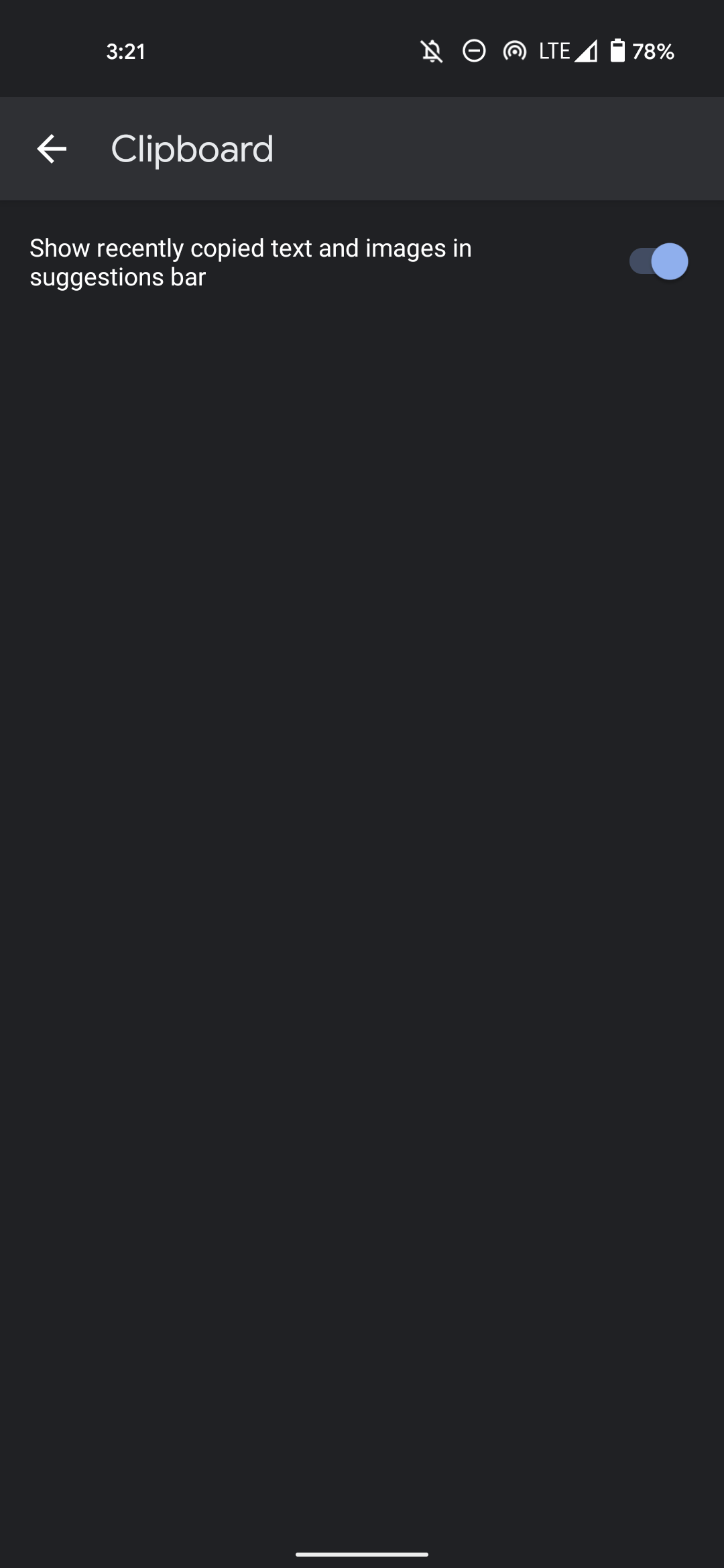The image displays a cell phone screen with a user interface related to clipboard settings. At the very top, typical cell phone indicators are visible, including the time, signal strength, type of network signal, battery charge, and other status icons. The background is a solid black, providing a stark contrast for the white text overlaid on it. Just below the status icons, there is a navigation bar labeled "Clipboard," featuring a left-pointing arrow, suggesting the option to return to a previous screen. Below the navigation bar, there is a blue slider button labeled "Show recently copied text and images in the suggestions bar," indicating that this feature is currently enabled. The rest of the page appears blank, with a small white bar at the bottom suggesting the end of the page's content.